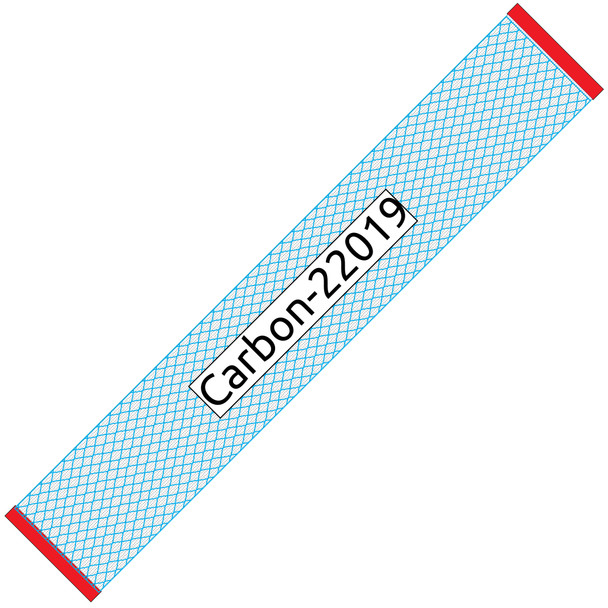The image features a long, thin, diagonal rectangle extending from the upper right-hand corner to the lower left-hand corner against a white background. At each end of this rectangle, there is a thin red strip. The main body of the rectangle consists of a blue and white diamond-shaped pattern. At the center of this patterned rectangle is a white label bordered in black, displaying the text "Carbon-22019" in black font. The rectangle is likely a label or sticker, with its blue and white pattern forming a grid-like appearance.